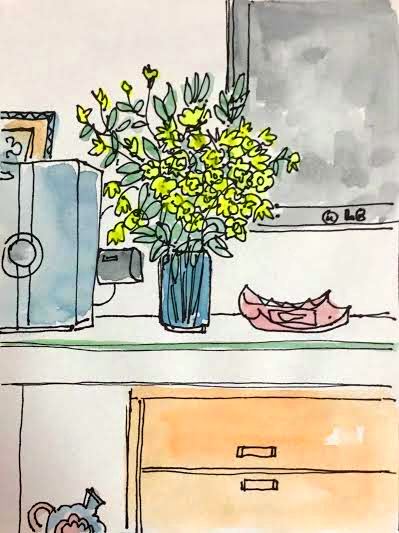This detailed illustration depicts a kitchen interior within a home. Mounted on the wall is a large gray appliance branded with the LG logo; its exact function is ambiguous, possibly a microwave or an unconventional fridge. On the counter below, there is an object that appears either as a plate with curved edges or a stack of papers. Nearby, a vase filled with vibrant, bright yellow flowers adds a pop of color to the scene. Another gray appliance, resembling a safe or perhaps a smaller countertop microwave, is also present. The kitchen is furnished with several brown drawers and closed cabinets. Lastly, a partially obscured framed picture hangs on the wall, peeking out from behind one of the gray appliances, contributing an artistic touch to the welcoming environment.